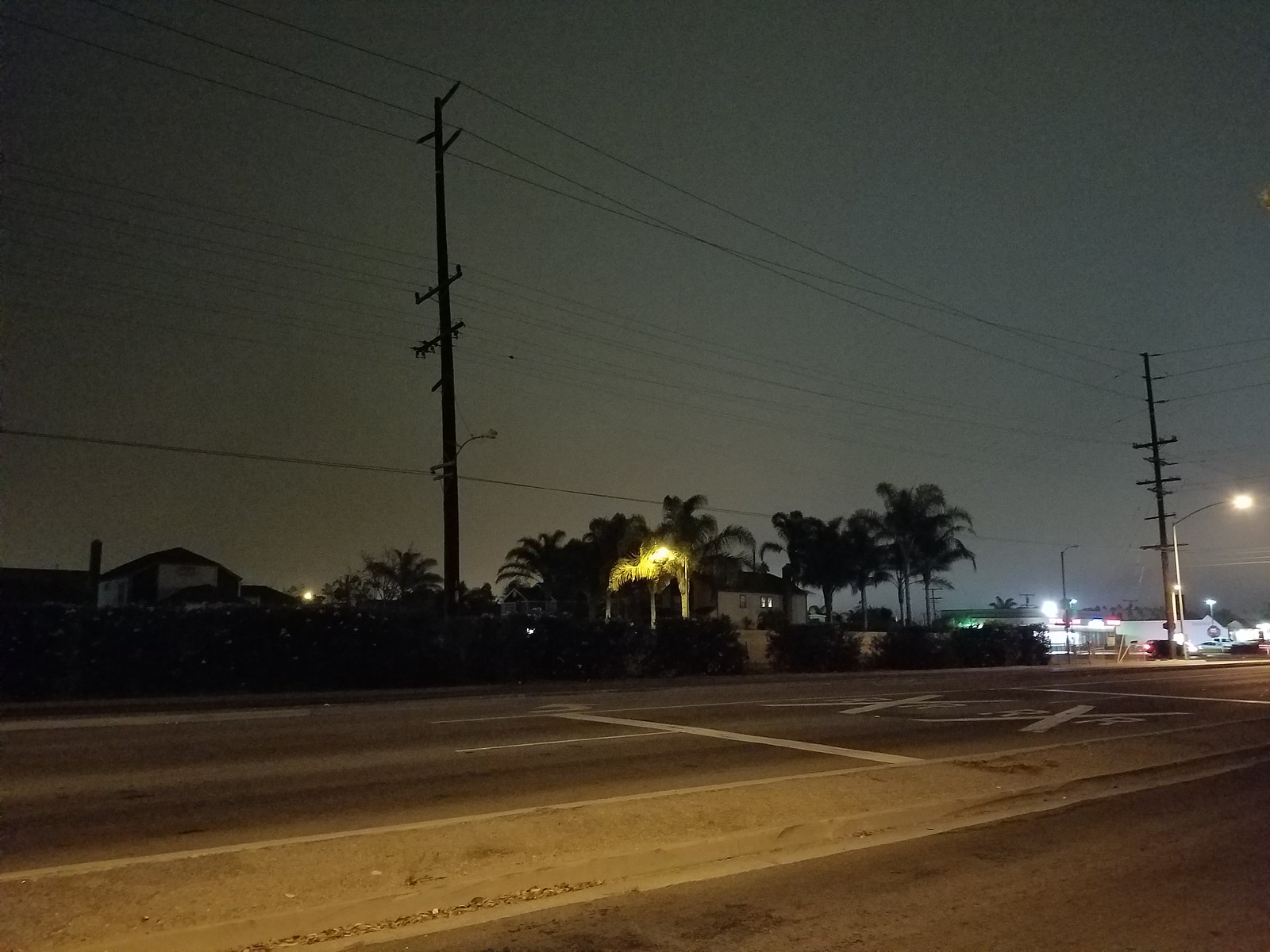A nighttime color photograph captures a serene, empty street scene. The image prominently features a one-story home in the background, subtly illuminated by a light to its immediate left. This light bathes several tall palm trees that both surround the building in the rear and grace its left side. Additional palm trees are visible in the foreground, positioned just left of the center of the frame.

A towering vertical utility pole stands prominently just left of center; it boasts three or four horizontal braces supporting multiple telephone, telegraph, and power lines. A similar utility pole is visible at the far right edge of the photograph, marking an intersection. Adjacent to this pole is a street lamp that casts a much brighter light, enhancing the visibility of that portion of the image. Far in the background, there appears to be a store or similar establishment, identifiable by a large, glowing light.

On the road, just right of center and toward the lower half of the frame, distinct white railroad crossing markings (X and two Rs) are painted, signaling an upcoming railroad crossing not visible in the shot. In the foreground, a concrete or cement traffic island enters the frame diagonally from the left, stretching up to the lower right edge before exiting out of view.

The sky above is a hazy black, adding to the quietude of the scene. The photograph, which contains no visible text or print, is well-focused, capturing an undisturbed moment free of any vehicles.